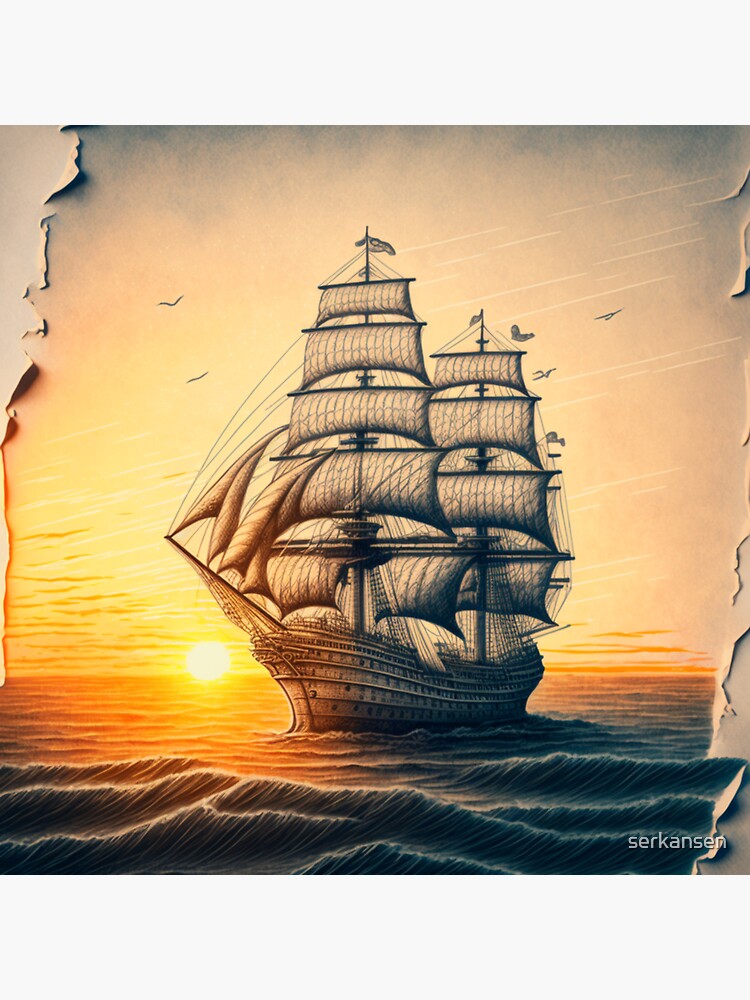The image is a detailed illustration, likely created with colored pencils or as a computer-generated line drawing, depicting a large wooden caravel-style ship in the ocean, possibly from the 1700s or 1800s. The ship, which resembles an old-fashioned pirate ship, features two masts with rows of large sails—five on the first mast and four on the second. The vessel is adorned with multiple rows of windows, possibly up to six, from top to bottom, and is shadowed in a dark blue hue. This significant detail emphasizes the ship's massive size. The scene is set against a vivid backdrop where the sun, either setting or rising, sits right on the horizon, casting a golden-orange glow over the expansive water and reflecting off the sky. Flocks of birds follow the ship as it journeys through slightly wavy waters. The illustration is remarkably well-crafted, although parts of it appear to be peeling away at the edges, revealing a plain, slightly brownish-gray tone beneath, adding a textured, almost weathered effect to the piece.